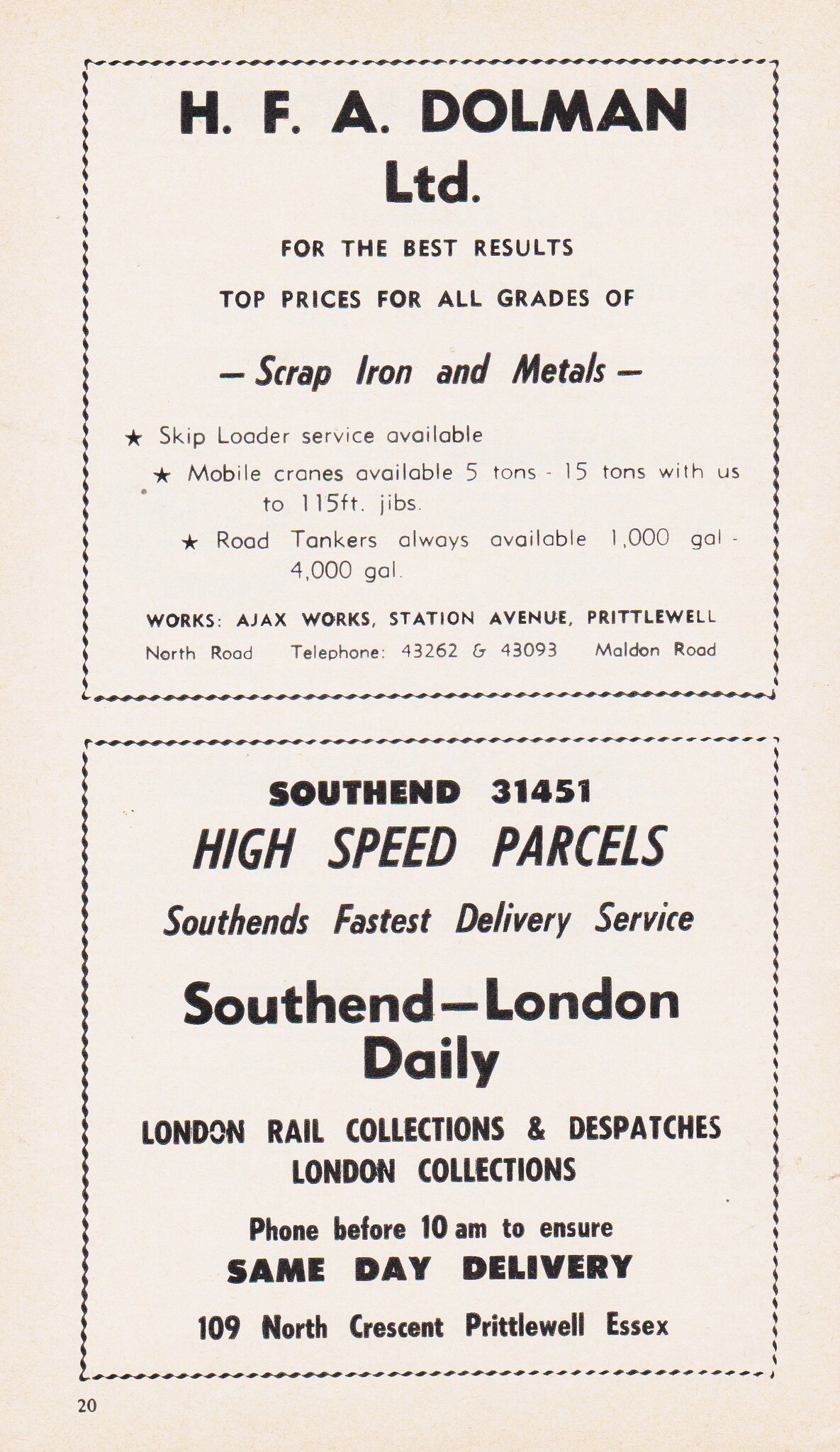The image depicts an old pamphlet, characterized by a large piece of pink paper, possibly indicating page 20 of a larger book, given the number '20' in the lower left corner. The paper is divided into two distinct squares with black boundaries.

In the top square, there is an advertisement for HFA Dolman Limited. It promotes their services related to scrap iron and metal, stating "For the best results, top prices for all grades of scrap iron and metals," implying they are buyers of such materials.

The bottom square features an advertisement for a high-speed parcel delivery service. It states: "South End 31451 High-Speed Parcels, South End’s Fastest Delivery Service." The ad details their services, which include daily deliveries from South End to London, rail collections and dispatches, and a note to phone before 10 a.m. to ensure same-day delivery. The address provided is 109 North Crescent, Pridwell, Essex.

Both advertisements reflect business services offered in the past, with the top square focusing on metal recycling and the bottom on expedited parcel delivery.